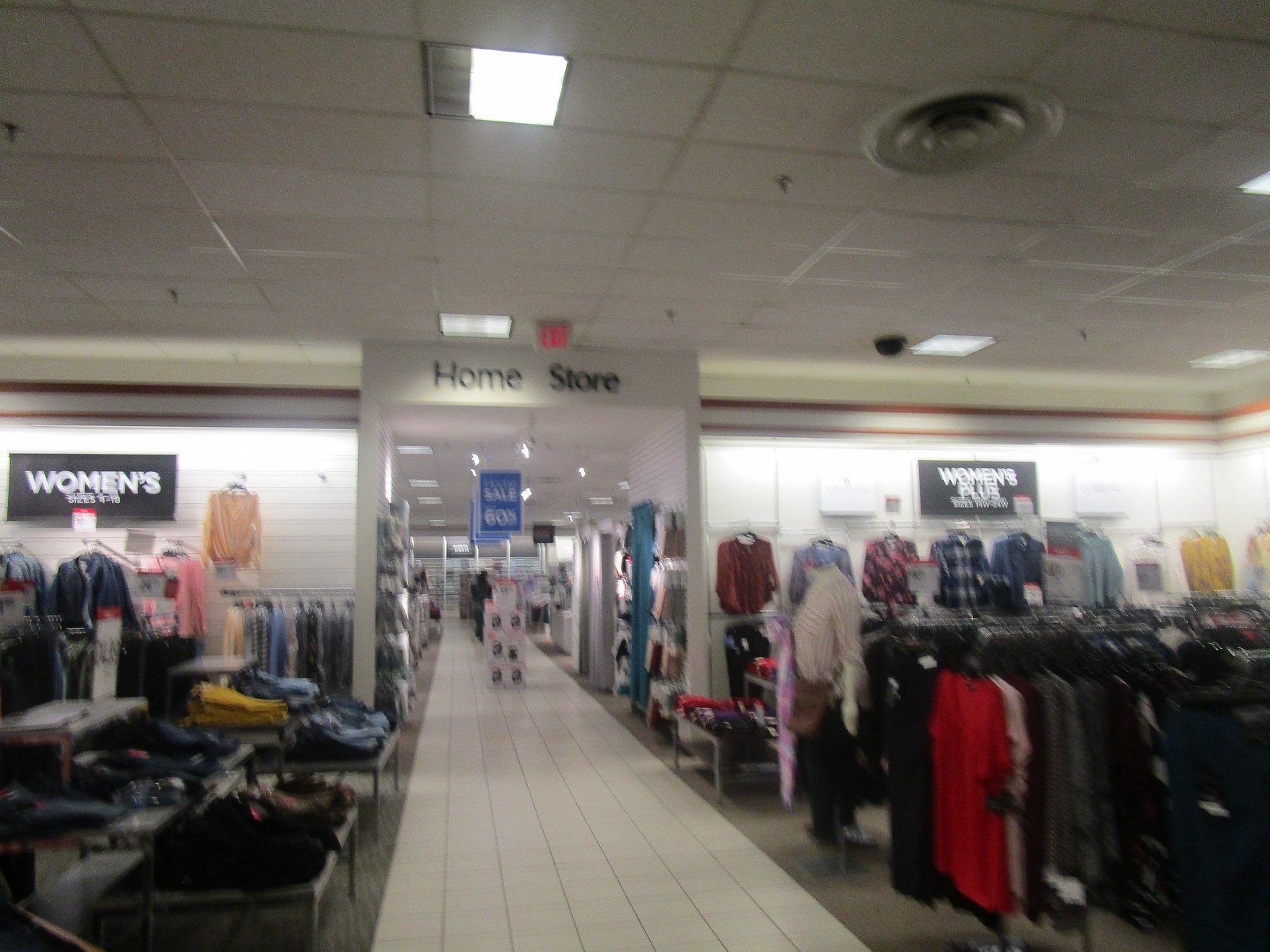In this highly detailed photograph of a department store’s clothing section, the focal point is divided into several distinct areas. In the upper left-hand corner, a black sign with white lettering designates the "Women's" section, while the upper right-hand corner features a similar black sign marking the "Women's Plus" section. A rectangular-shaped opening in the background leads to another area of the store labeled "Home Store" with a prominent blue sign announcing a "Home Sale 60% off." This entry is crowned with a red exit sign.

The right-hand side of the image showcases metal hang rods laden with diverse clothing items, including various patterns and solid colors in whites, browns, grays, reds, pinks, and yellows. Notable among the displayed items is a mannequin modeling an outfit. In contrast, the left-hand side features a similar array of clothing, but here the garments are arranged on tiered tables rather than hanging rods. Jeans and other folded items are visibly laid out on these counters.

The middle of the aisle is marked by tile flooring leading into the "Home Store" section where additional items like curtains and slippers are visible. Overall, the scene encapsulates the organized yet bustling atmosphere typical of a department store, with an emphasis on women’s fashion and home goods.